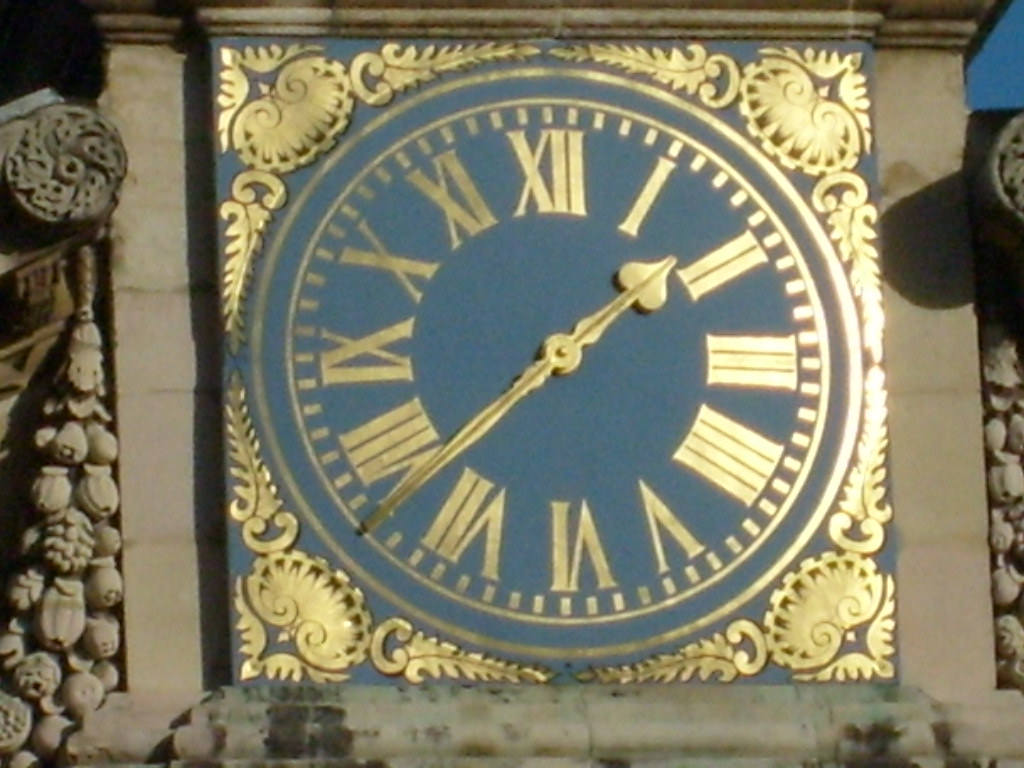The image features a photograph capturing a striking clock prominently emblazoned with gold letters, numbers, and trim. The clock stands out against a very light blue background, creating a vivid contrast. The centerpiece of this clock rests on two sturdy concrete pillars, which are a grayish-beige cement color. On the left side of the image, intricate flower motifs are embedded within the concrete pillar, adding a touch of elegance and detail. The right side reveals a glimpse of the bright sky, suggesting the photograph was taken during the daytime. The overall brightness of the image enhances the richness of the gold accents and the fine details in the floral concrete designs.